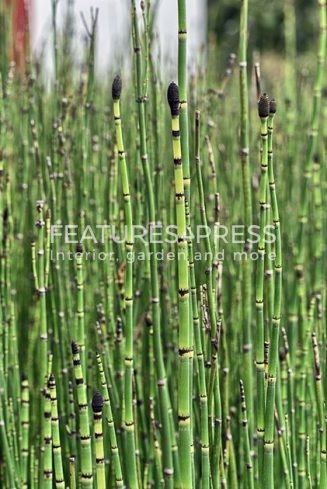The image depicts a densely packed outdoor setting filled with tall, slender green stalks resembling bamboo or asparagus, each segmented with a black tip or pod at the top. These stalks occupy three-quarters of the photograph, creating a dominant visual element. The blurred background features what appears to be a white shed positioned towards the left side. Overlaying the bottom and middle sections of the image is a transparent text layer that reads "Features, Press, Interior, Garden, and More" in a grayish font. This combination suggests that the image might be a cover for a book, advertisement, or magazine, emphasizing the aesthetic appeal of the garden environment highlighted by the orderly, bamboo-like plants.